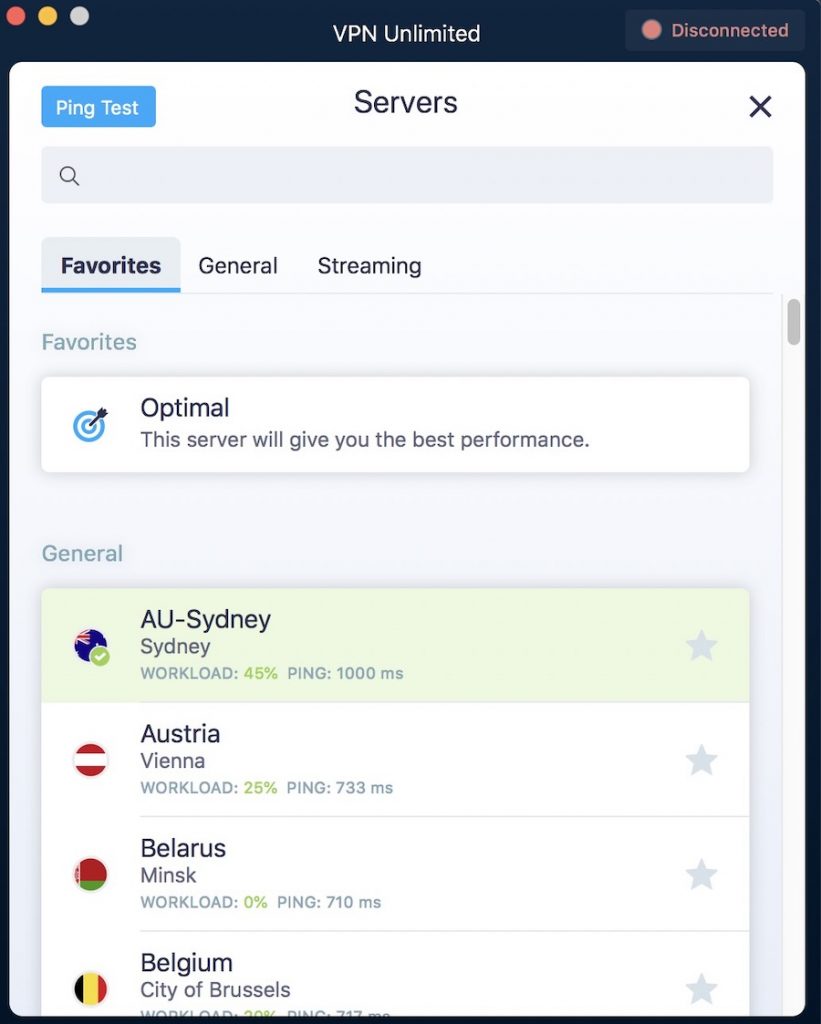This screenshot captures the interface of a VPN app displayed on a Mac. In the top left corner, the typical Mac window controls—close, minimize, and maximize—are visible. The top row prominently features the title "VPN Unlimited" in the center. On the right side of this row, the status "Disconnected" is indicated with a red circle. 

Directly below, there is a "Servers" section with a "Ping Test" blue button on the left and a close window "X" on the right. Beneath this row is a search box for locating servers. 

The user is currently viewing the "Favorites" tab, which is one of three tabs available—Favorites, General, and Streaming. In the "Favorites" tab, a highlighted box labeled "Optimal" suggests this server will deliver the best performance.

Under the "General" section, four server locations are listed:
1. **AU-Sydney**: Workload at 45% and a ping of 1000 milliseconds.
2. **Austria, Vienna**: Workload at 25% and a ping of 733 milliseconds.
3. **Belarus, Minsk**: Workload at 0% and a ping of 710 milliseconds.
4. **Belgium, Brussels**: The workload and ping times are not clearly visible.

Overall, the user interface is neatly structured, providing intuitive options for connecting to various VPN servers efficiently.